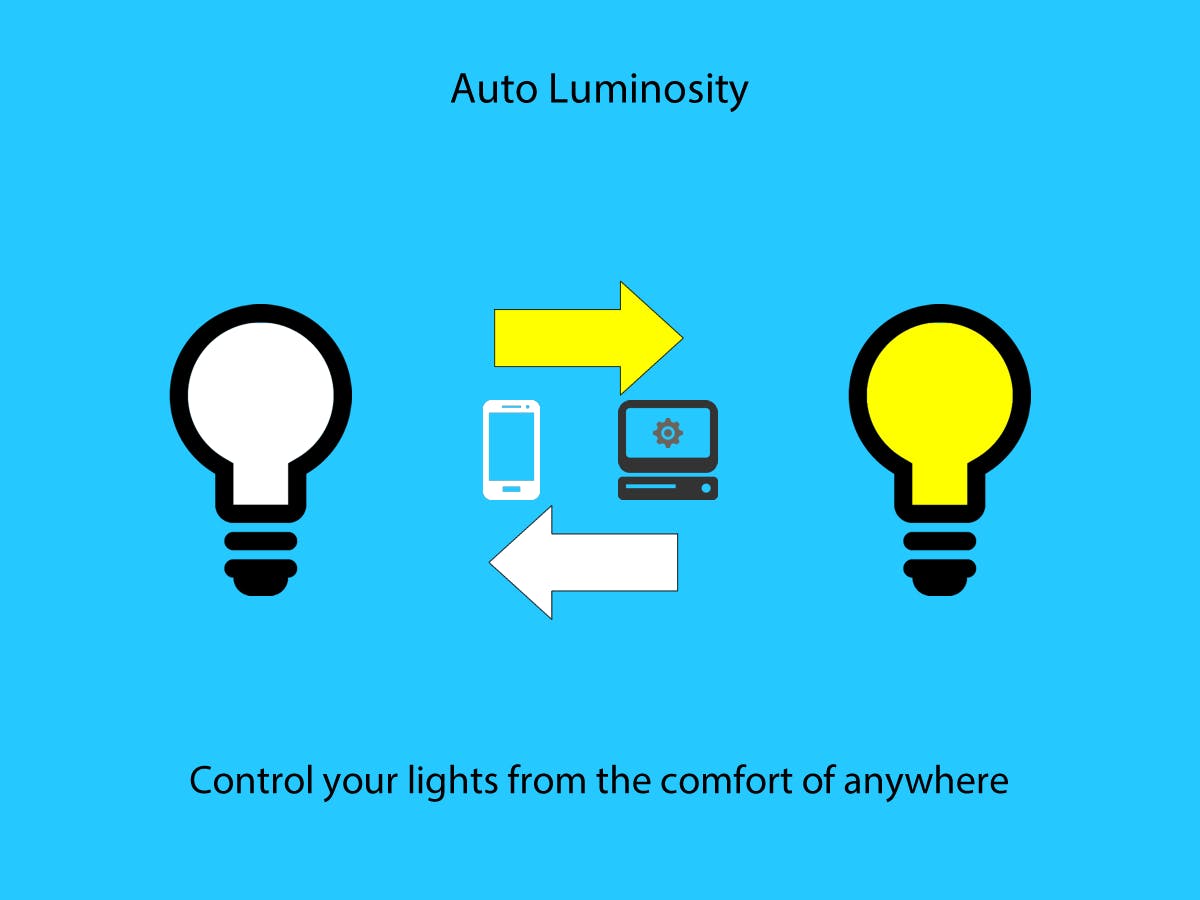The image appears to be an advertisement promoting an environmentally friendly control system for lights, emphasizing the concept of "auto-luminosity." The ad features a baby blue background with black text at the top that reads "Auto Luminosity." It also includes the slogan, "Control your lights from the comfort of anywhere," written in black at both the top and bottom of the ad.

Two light bulbs, one white and one yellow, are positioned on the left and right sides of the image. Yellow and white arrows point between the light bulbs, indicating a change in lighting or connectivity. The center of the image depicts icons of a cell phone and a computer, suggesting that the lights can be controlled remotely through these devices. The predominant colors in the ad are yellow, white, black, and blue. This ad is likely created by a company promoting environmentally considerate solutions for lighting control.